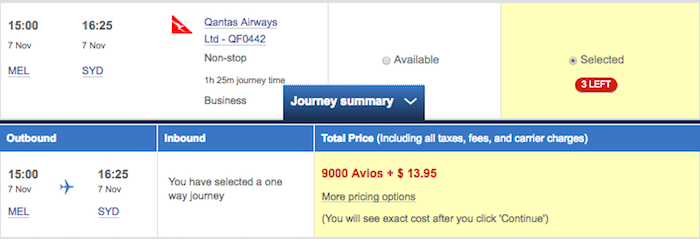A detailed, cleaned-up caption for the described image could be:

---

The image showcases a travel airline booking site displaying search results for a round-trip flight from Melbourne (MEL) to Sydney (SYD) on November 7. The first available flight is with Qantas Airways, indicated by the prominent Qantas logo featuring a red triangle with a kangaroo. This flight, QF0442, departs at 1500 hours from Melbourne and arrives in Sydney at 1625 hours, offering a non-stop journey of 1 hour and 25 minutes with business class options. A highlighted notification indicates that only 3 seats are left. 

In the center of the screen, a tab labeled "Journey Summary" on a blue background details the trip's itinerary. The summary includes "Outbound" and "Inbound" sections and conveys the total price including all taxes, fees, and carrier charges. The outbound journey details are repeated, with icons representing the flight path. The inbound section denotes that the selected journey is one-way. The total cost is boldly presented in red as "9,000 AVOs plus $13.95." 

Below, there's a link option for more pricing choices, with a note that exact costs will appear upon continuing the booking process. This information is within a yellow-highlighted field. The section ends with a gray line at the bottom, with no additional details following it.